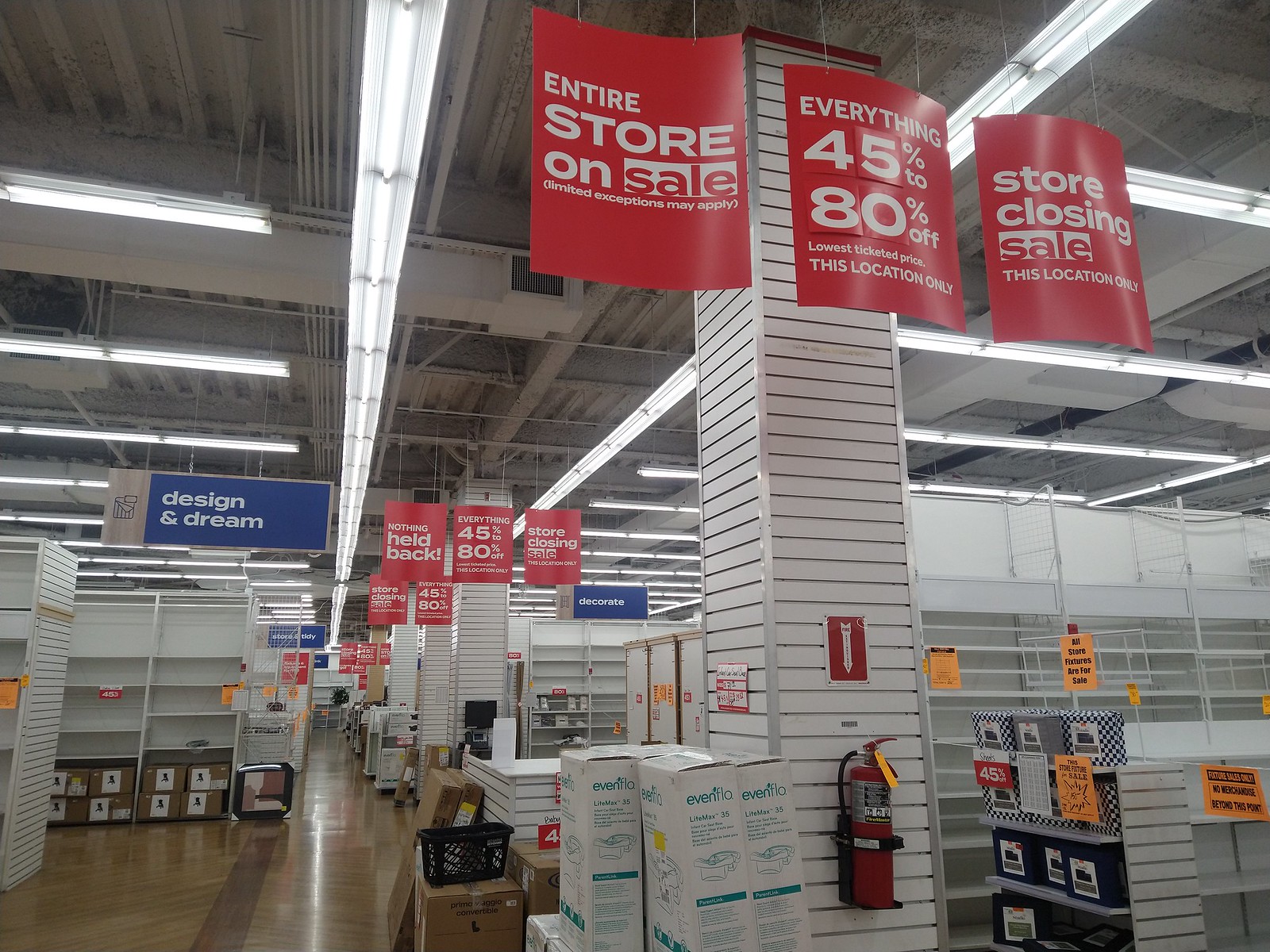The interior of a department store is detailed in this image, characterized by a predominantly gray ceiling. A strip of fluorescent lighting runs on both the left and right sides of the ceiling. In the middle, a structural support beam extends from the front to the back of the store. Mounted along this beam are multiple white boards that rise and fall in a rhythmic pattern.

Below, an array of white metal shelves stretches toward the back of the store, creating a sense of depth and organization. At the top of the image, three banners are prominently displayed. The first banner announces, "Entire Store on Sale." The second banner reads, "Everything from 5% to 8% Off, This Location Only." The third banner declares, "Store Closing Sale," highlighting the store's final sales event. Despite the sale, several items remain in the store, as evidenced by the still-stocked shelves and multiple signs indicating ongoing promotions. The overall scene suggests an atmosphere of urgency and transition as the store prepares to close its doors permanently.